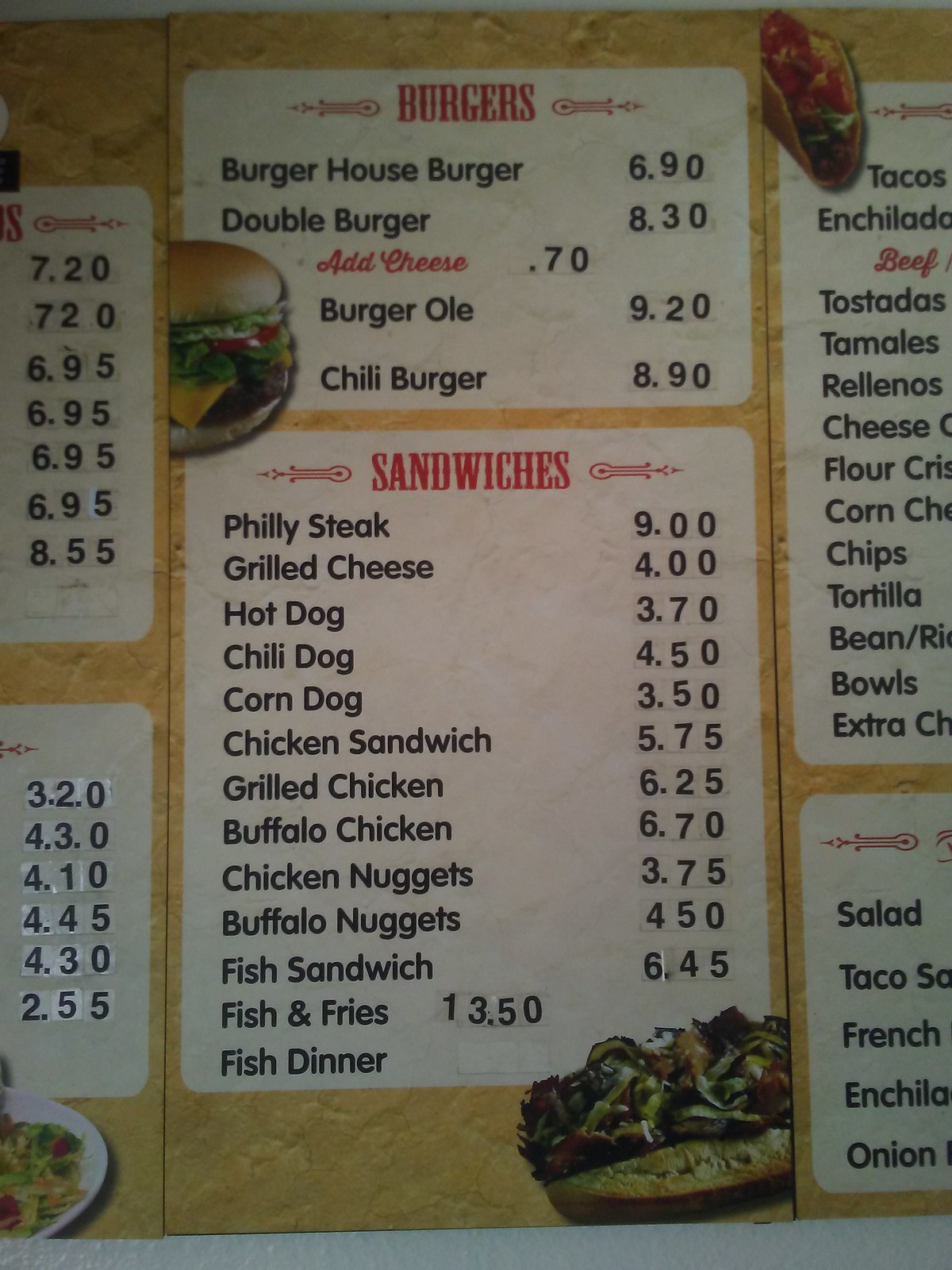This image captures a close-up view of a brightly colored menu mounted on a wall. The menu is predominantly red and white with yellow highlights, and it seems to cater to a casual dining experience, likely a diner or fast-food setting. The menu is divided into two main sections: "Burgers" and "Sandwiches."

In the "Burgers" section, located at the top half of the menu, the listed items are as follows:
- House Burger: $6.90
- Double Burger: $8.30
- Add Cheese: $0.70
- Burger Olay: $9.20
- Chili Burger: $8.90

The "Sandwiches" section occupies the bottom half of the menu and includes a wide variety of options:
- Philly Steak
- Grilled Cheese
- Hot Dog
- Chili Dog
- Corn Dog
- Chicken Sandwich
- Grilled Chicken
- Buffalo Chicken
- Chicken Nuggets
- Buffalo Nuggets
- Fish Sandwich
- Fish and Fries
- Fish Dinner (price not listed)

Each section features corresponding images to enhance the clarity of the offerings. A picture of a burger is situated near the burger section, a taco image is nearby for context (perhaps indicating other menu items not listed), and a sandwich picture is placed at the very bottom associated with the sandwich options. The vibrant colors and straightforward layout make it easy for customers to navigate and select their preferred items.